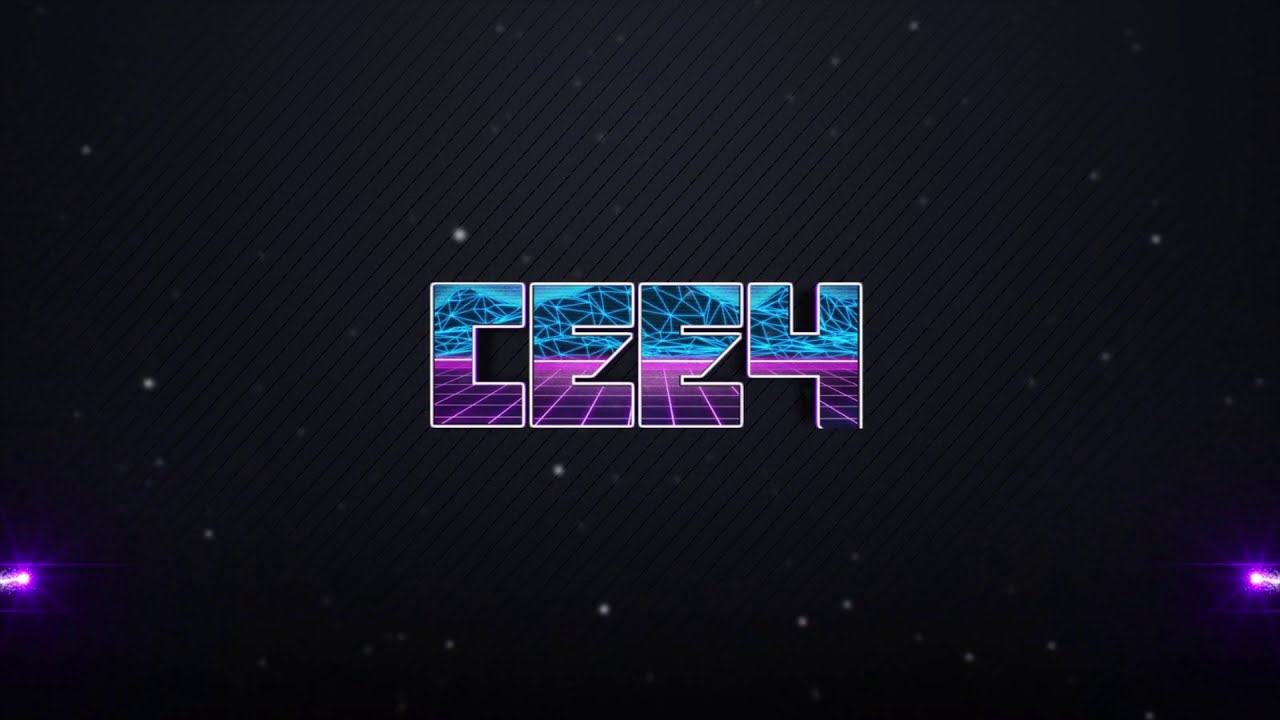The image is a captivating depiction of a futuristic and possibly outer space theme with a predominantly black background, overlaid with horizontal stripes of an even darker black, extending from the bottom left to the top right corner. Scattered throughout the background are indistinct, blurry white orbs, reminiscent of distant stars. In the center, large stylized block letters reading "C.E.E.4" command attention, split by a white dividing line. The top halves of these characters showcase a blue design featuring black mountains intertwined with glowing blue lines, while the bottom halves display a vibrant purple grid pattern. The text characters are bordered in white, enhancing their prominence. Adding to the animated effect, the bottom left and right edges of the image have vibrant purple glowing elements protruding from the sides. The overall aesthetic suggests it could be an advertisement for a video game set in a futuristic or outer space setting.